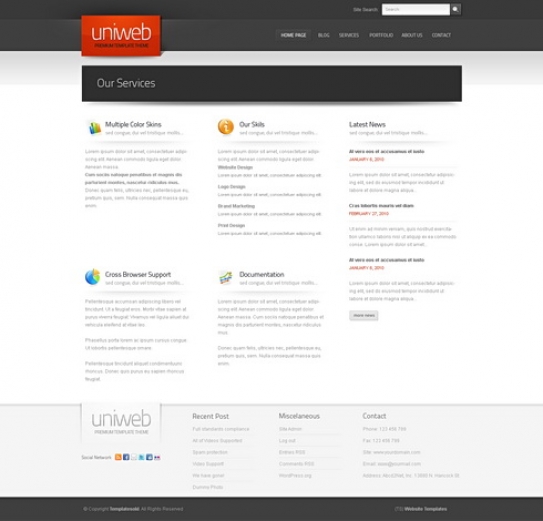Caption:
"Introducing 'Uniweb,' prominently displayed in a white font within a red rectangular box. Beneath the name is a tagline that, although too small to read, hints at the brand's mission. This part of the image rests on a sleek black background, contrasting with the main page's clean white canvas. The main page hosts various sections including 'Our Services,' 'Multiple Color Skins,' 'Cross-Browser Support,' 'Our Skills,' 'Documentation,' and 'Latest News,' likely comprised of brief blog entries. At the bottom, there's an array of contact information and social media links for easy connectivity. A search bar is conveniently located at the top right, alongside main navigation sections labeled 'Homepage,' 'Blog,' 'Services,' 'Portfolio,' 'About Us,' and 'Contact.' Despite the finer details of the text being unreadable, the overall layout suggests Uniweb is an all-encompassing platform designed to help users create compatible, customizable websites with ease."